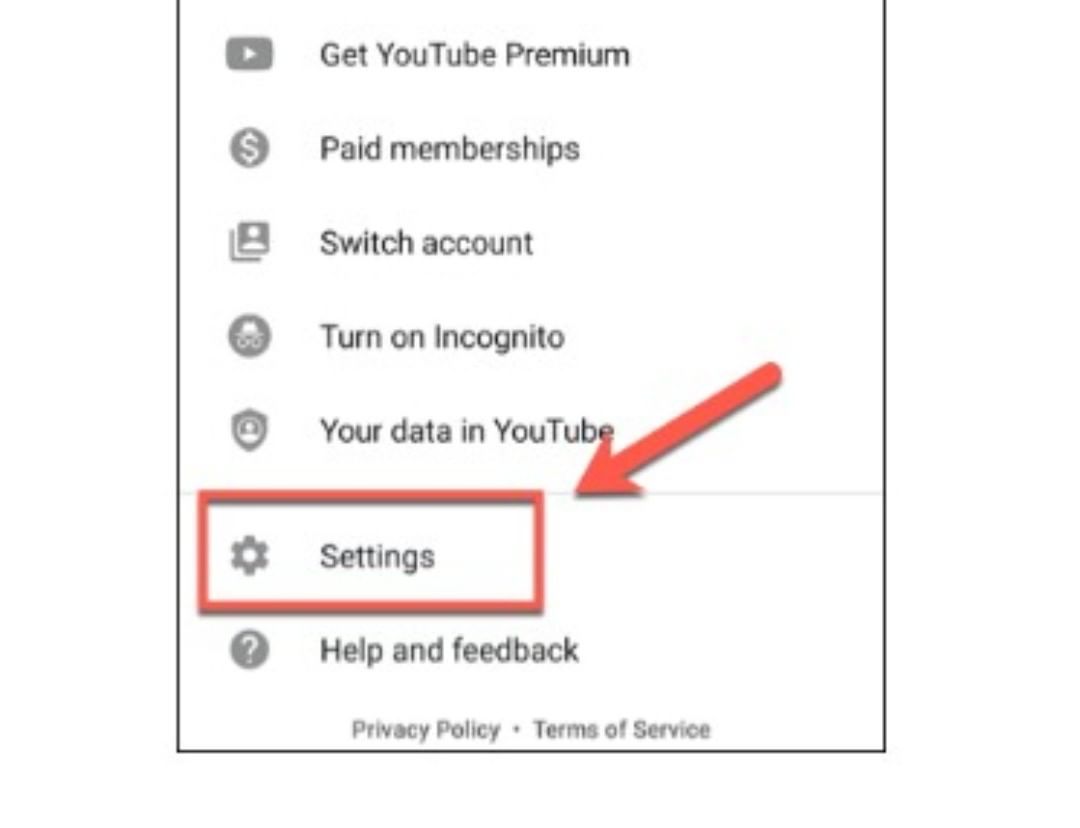In this image, you can see the settings menu of the YouTube interface. At the top left corner, there's the YouTube logo followed by the text "Get YouTube Premium." Below this, there is a list of menu options in gray text accompanied by gray icons. The first option displays a coin symbol and reads "Paid memberships." Following that, the menu options listed are "Switch account," "Turn on Incognito," "Your data in YouTube," a dividing line, "Settings," and "Help and feedback." A red rectangle highlights the "Settings" option, and a red arrow in the upper right corner points towards this highlighted box. At the bottom of the menu, you can see the words "Privacy," "Terms," and "Service." Although the image is slightly blurry, the text and icons are still legible and aligned vertically.